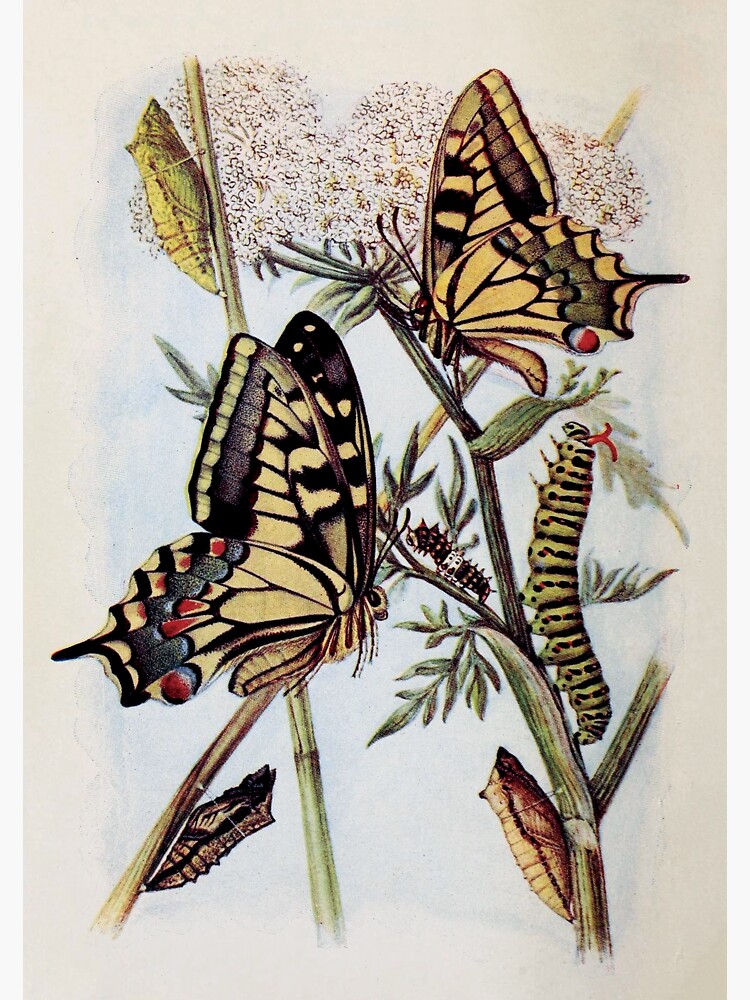In this detailed illustration, we see various stages of a butterfly's life cycle represented along a green plant stem against a light gray backdrop. At the top left, a lime-green chrysalis is attached to the tip of the stem, signifying the pupa stage. Below this, there is a vibrant butterfly with goldish-yellow wings, embellished with black and red details. Its body is yellow with black antennae and eye, and it features a distinctive red circle at the bottom of its wings. Directly opposite this butterfly, another yellow butterfly mirrors its appearance with similar black, red, and yellow patterns, though it is viewed from the side. Beneath this second butterfly, a green caterpillar with black streaks and red antennae stands vertically. Toward the bottom of the stem, further diverse insect life is depicted, including a couple of unidentified brown and black bugs. The plant itself boasts a mix of green stems and flowers that appear to be white-spotted, possibly resembling dandelions. The detailed painting captures the animated ascent of each insect, emphasizing a sense of upward movement through the intricate depiction of each life stage.